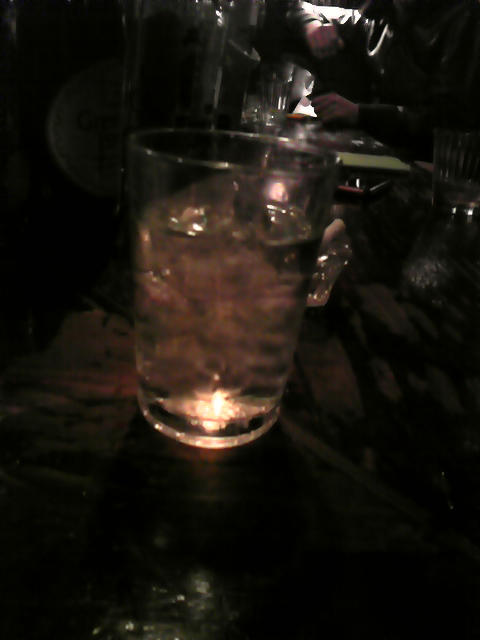The photograph captures a dark and moody bar scene primarily focused on a glass with a handle, resembling a mug, filled with a clear liquid that takes on a pink tint due to a light source shining from behind. This illumination bounces off the bottom of the glass, casting an ethereal glow that creates an eye-catching focal point amidst the pervasive darkness. The table it rests on is brown, contrasting with the largely black surroundings which include dark walls and another black table visible in the background. 

In the rear, partially visible through the shadows, is a man wearing a black long-sleeve shirt and what appears to be a necklace. His face is obscured due to the low lighting, but his hand on the table can be made out. Other details include additional glasses, a phone, and a light yellow piece of paper scattered on the table. Further into the background, about 20 feet away, there seems to be other patrons indistinctly visible, adding depth to the scene. A white circular sign with some text in the top left corner faintly stands out, completing the dimly lit bar ambiance.